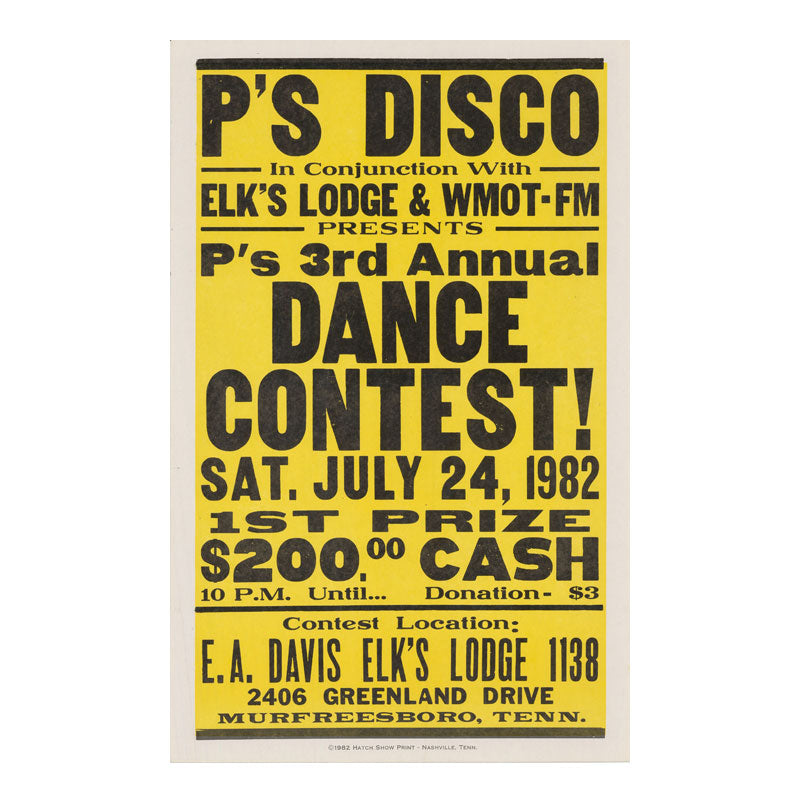The image showcases a vibrant yellow poster with a bold black font, bordered by off-white edges and highlighted by black lines at both the top and bottom. The poster prominently advertises "P's Disco in conjunction with Elks Lodge and WMOT-FM presents P's 3rd Annual Dance Contest." The event is scheduled for Saturday, July 24, 1982. The grand prize for the contest is $200 cash. The event starts at 10 PM and continues until the late hours, with a suggested donation of $3 for entry. The contest will be held at the E.A. Davis Elks Lodge, located at 1138, 2406 Greenland Drive, Murfreesboro, Tennessee. The text on the poster is strictly in black with no accompanying images, emphasizing the key details of the event.